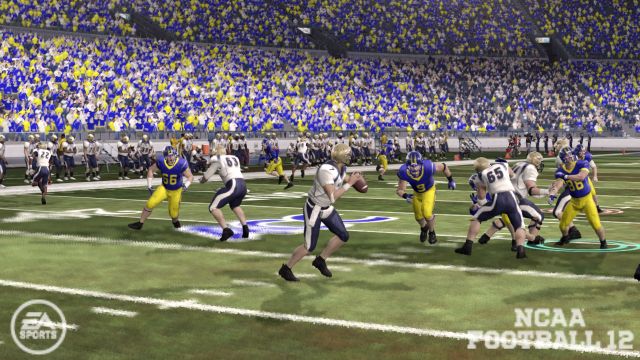The image captures an intense moment from a football game, viewed from a slightly elevated position behind and to the right of the quarterback, who is poised to throw the ball. In the foreground, the quarterback's stance and focus are evident, encapsulating the action and anticipation of the play. The center of the image showcases the football field with several players positioned and ready for the next move, highlighting the strategic nature of the game. The backdrop features a two-tiered stadium filled with animated spectators, adding to the vibrant atmosphere of the event. The lower left corner of the image displays the EA Sports logo in a white, bold font within a white circle. On the bottom right, the text "NCAA Football 12" is prominently featured in white font, denoting the title of the game.